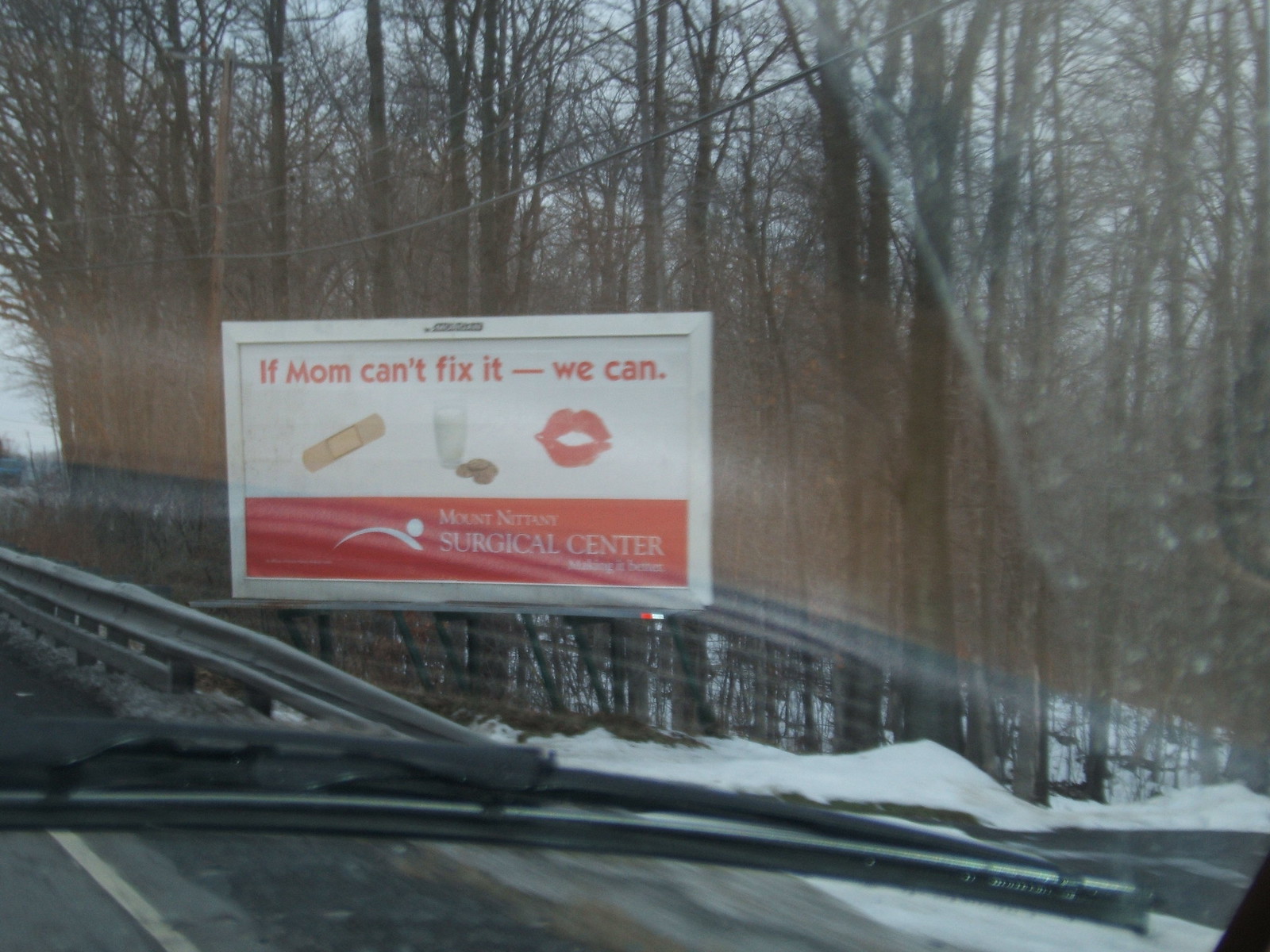The image, taken through the windshield of a car, captures a small billboard on the side of a snowy highway. Prominently featuring the windshield wiper spanning the lower portion of the scene, the winter setting is evident from the snow lining the road and the forested background with barren trees. The road's white edge stripe and guardrail indicate it's a highway. The rectangular, horizontally oriented billboard, situated left of center, has a white upper two-thirds and a red lower third. In red letters across the top, it reads, "If Mom Can't Fix It, We Can." A colorful band-aid adorns the left side, while the center showcases a glass of milk and a stack of chocolate chip cookies, accompanied by a lipstick kiss mark, presumably from a mom. The bottom red section bears the text, "Mount Nittany Surgical Center," in white lettering.